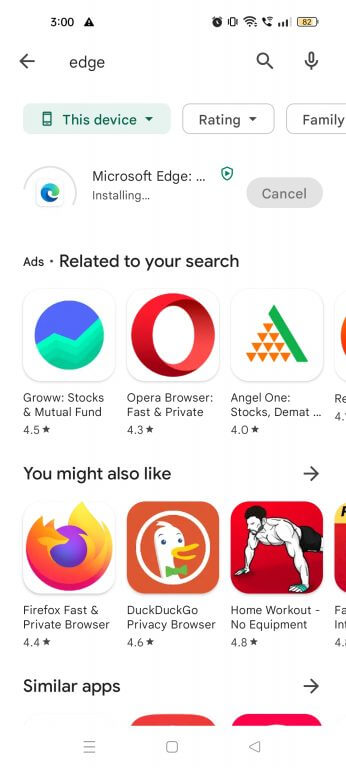A smartphone screenshot showcasing a detailed interface. In the upper right corner, a battery indicator is visible, while the upper left corner displays the current time. Between these are various function icons related to the telephone. The focus is on a search query for "Edge," which has been input into the phone's search bar. The results show a hyperlink for Microsoft Edge, with a status update indicating that the application is currently installing. Below this, there is a section labeled "Ads related to your search," displaying several app logos. Each app logo is accompanied by its name in a dark blue or black font and a star rating, offering additional app options beyond Microsoft Edge.